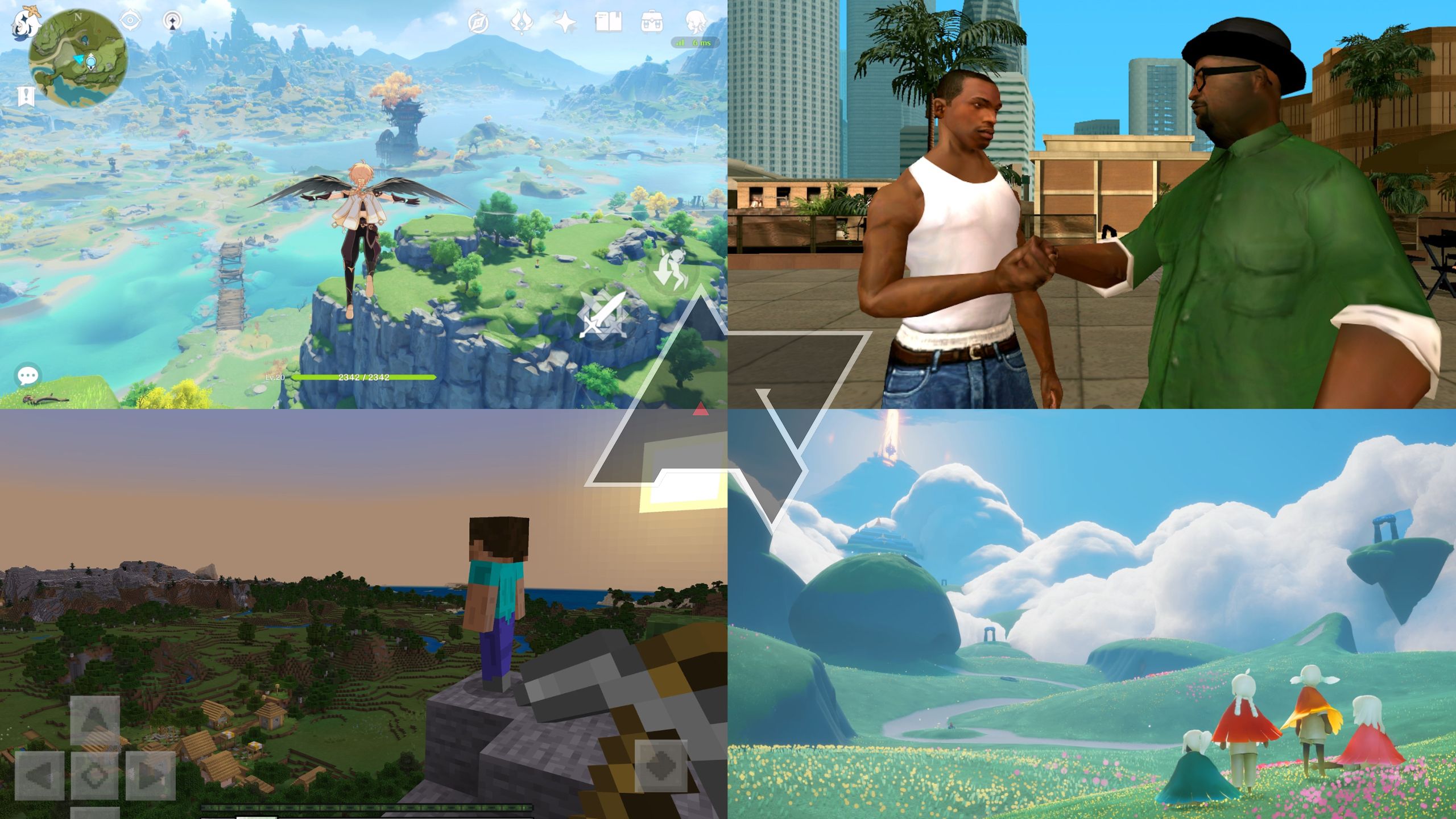The rectangular horizontal image is divided into four quadrants, each containing distinct imagery indicative of video game and animated art styles. In the upper left quadrant, a painted or cartoon character with angel wings soars over an expansive scene with mountains, water, and greenery. The character is dressed in a white top and black pants. Moving to the upper right, two individuals, likely African-American men, are engaging in a handshake or fist bump. One man is wearing a green shirt and a hat, while the other wears a white tank top and jeans, and they stand against an urban backdrop. The bottom left quadrant depicts a blocky, pixelated character reminiscent of Minecraft, standing on a ledge overlooking a verdant valley. Finally, the bottom right features a whimsical scene with a couple, both in white hats and red capes, standing with two children dressed in a red dress and green cape, respectively. They are gazing at a picturesque cloud formation against rolling green hills. A logo resembling "A7" can be seen in the middle, and the upper left quadrant has a little circle that might depict a pause button.